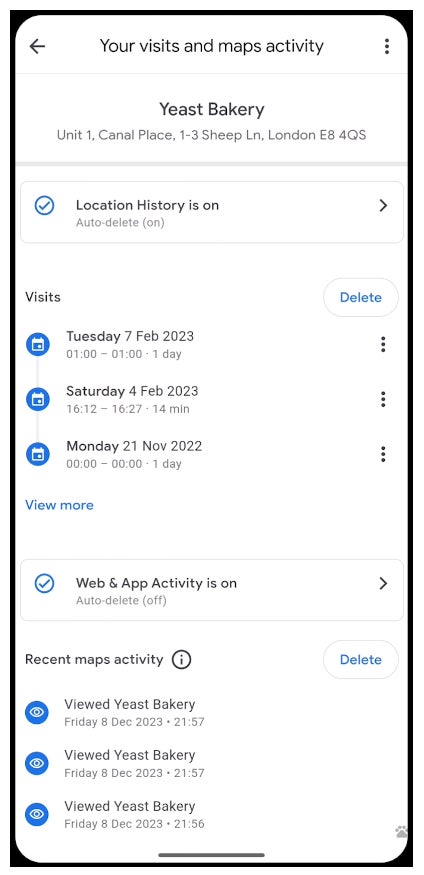This image, captured on a smartphone screen, details a user's location and activity history within a mapping application. The top section displays a summary under the heading "Your Visits and Maps Activity." The highlighted location is "Yeast Bakery," situated at Unit 1, Canal Place, 123 Sheep Lane, London, with the specific postal code provided. The text indicates that location history is enabled with an option for auto-deletion in progress.

The "Visits" section meticulously logs recent site visits, starting with Tuesday, February 7th, 2023, indicating the user spent one day at the bakery. There is a delete button and a three-dot menu offering additional options. Similarly, the log notes a visit on Saturday, February 4th, 2023, which lasted 14 minutes, and another visit on Monday, November 21st, 2022, for one day. A prominent "View More" link in blue, clickable font invites the user to access further historical data.

The subsequent section, titled "Web and App Activity," confirms that activity monitoring is active and features settings for auto-deletion, which can be toggled off via an arrow icon. This is followed by "Recent Maps Activity," accompanied by a large delete button. The user appears to have viewed "Yeast Bakery" three times on December 8th, as thrice documented consecutively.

Overall, the screen provides a comprehensive and interactive overview of location and activity records, with multiple tools for user management and data privacy.